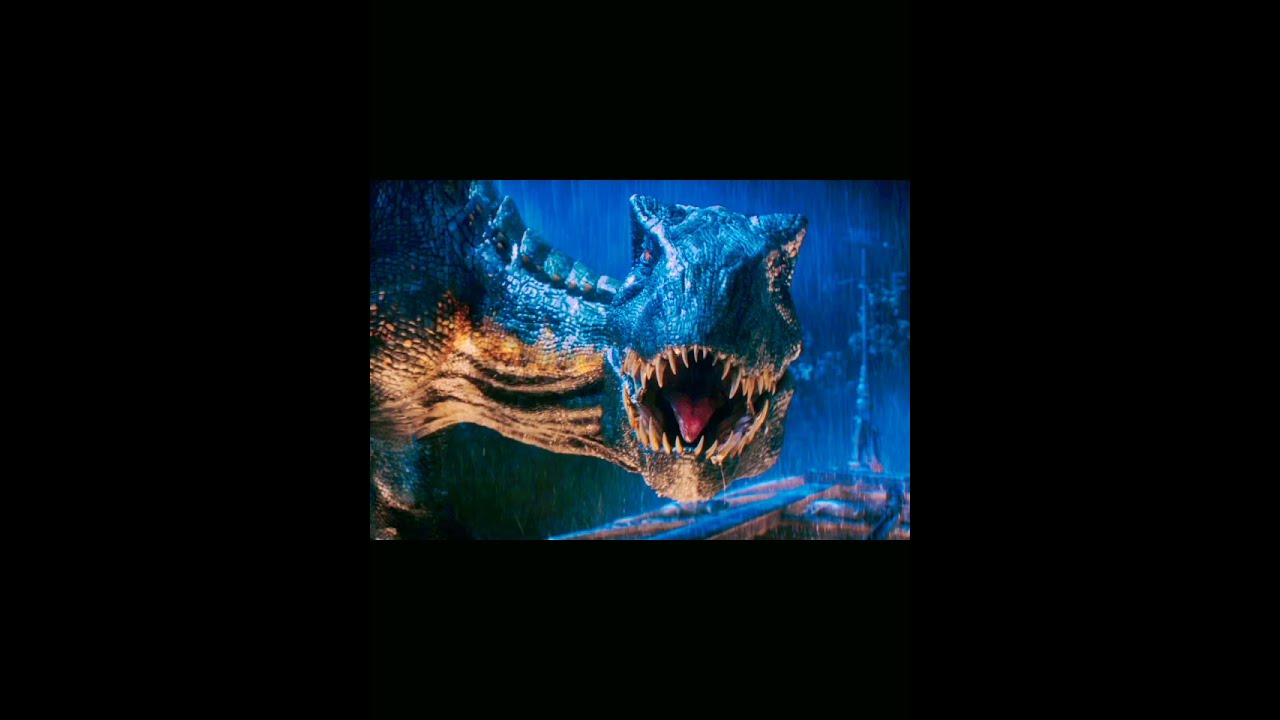The image is a detailed, close-up artwork of a massive, prehistoric Tyrannosaurus Rex, centered within a large, pure black background. The T-Rex, with bluish-green scales and yellow highlights, fills the center of the frame with its head and thick neck prominently displayed. The dinosaur's mouth is open, showcasing several sharp teeth and a large, red tongue, while its piercing eyes stare aggressively at the camera. The T-Rex is leaning down, with most of its body cropped out, extending out from the left side of the image. The scene appears to be set at night, with a dark blue to black backdrop and heavy rain pouring down. In the background, a metal tower and a wooden dock are visible, adding depth and context to the setting, giving the impression of a movie or video game scene. The overall atmosphere of the image is intense and ominous, with the rain and dark tones enhancing the fierce presence of the T-Rex.